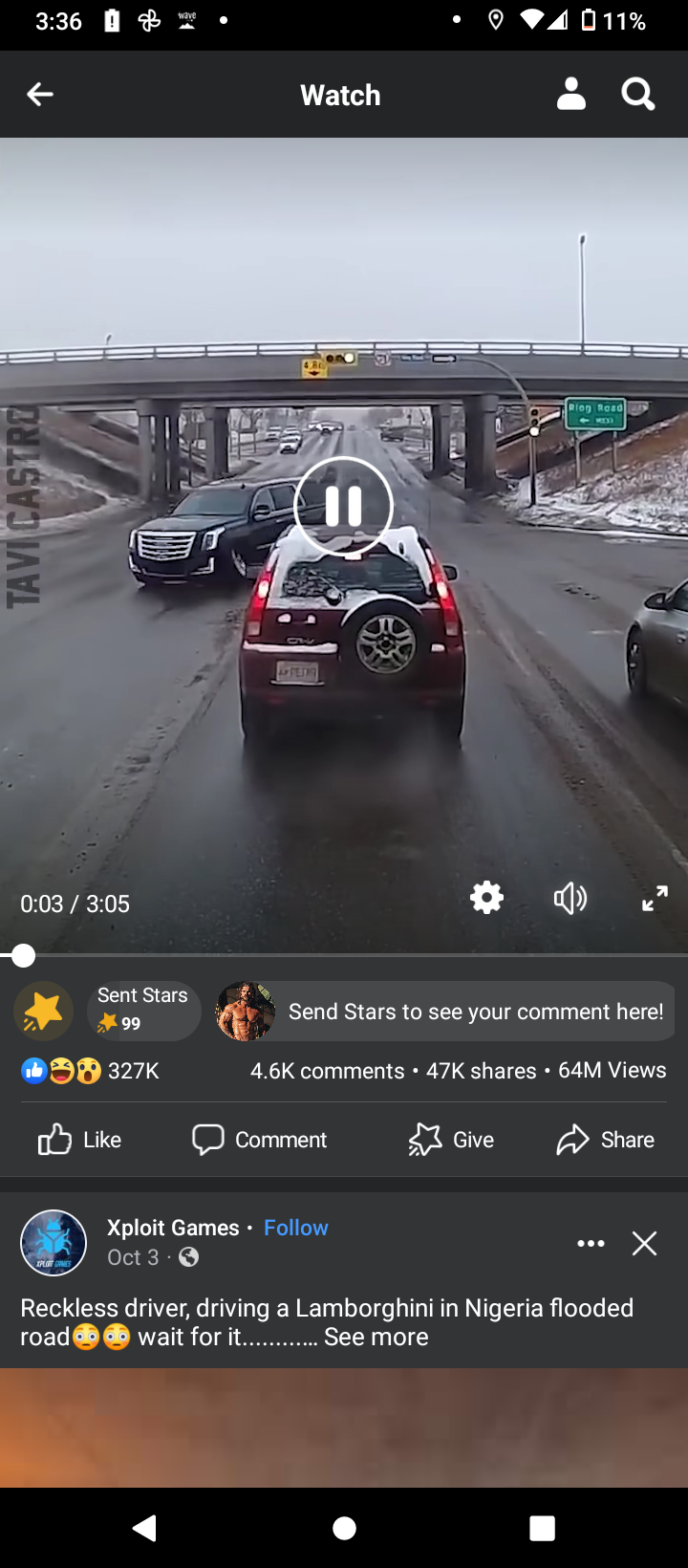This image is a screenshot from a smartphone, displaying a paused video on a social networking platform, likely TikTok or Facebook. At the very top, familiar smartphone icons are visible: the time is 3:36, the Wi-Fi is connected, and the battery level is critically low at 11%. Just below these icons, a gray strip reads "watch," indicating an active video.

The video itself shows a scene from a U.S. interstate highway. The perspective suggests the viewer is situated in the middle lane of a three-lane road. Directly ahead, a red car is visible, driving towards an overhead bridge in the distance. To the right side of the road, a green highway sign is posted, although the text is too small to read clearly in the screenshot. The overall scene captures a typical moment on a busy highway, emphasizing the digital and real-world intersections in our daily lives.